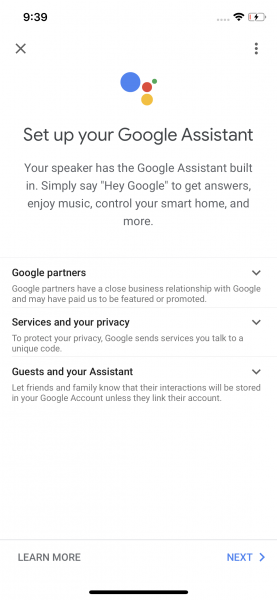The image depicts a screenshot taken from a smartphone showing the setup screen for Google Assistant. At the top, a message prompts the user to "Set up your Google Assistant," accompanied by a paragraph explaining the features available. The paragraph reads: "Your speaker has the Google Assistant built in. Simply say 'Hey Google' to get answers, enjoy music, control your smart home, and more."

In the upper-right corner of the screen, the current time is displayed as 9:39. Nearby, an 'X' icon allows the user to exit the setup screen. The battery icon shows it is charging, evidenced by a lightning bolt symbol and a slight yellow section on the otherwise white battery indicator. Additionally, three vertical dots on the right side signify a menu option.

Scrolling down, there's a section titled "Google Partners," describing Google's close business relationships and mentioning that some partners may have paid to be featured or promoted. Another section labeled "Services and Your Privacy" explains that Google assigns a unique code to services you interact with to protect your privacy.

Following that, the "Guest and Your Assistant" section advises users to inform friends and family that their interactions with the assistant will be stored in the user's Google account unless they link their own accounts. Below all these sections, options to "Learn more" and a blue "Next" button are visible, guiding users through the setup process.